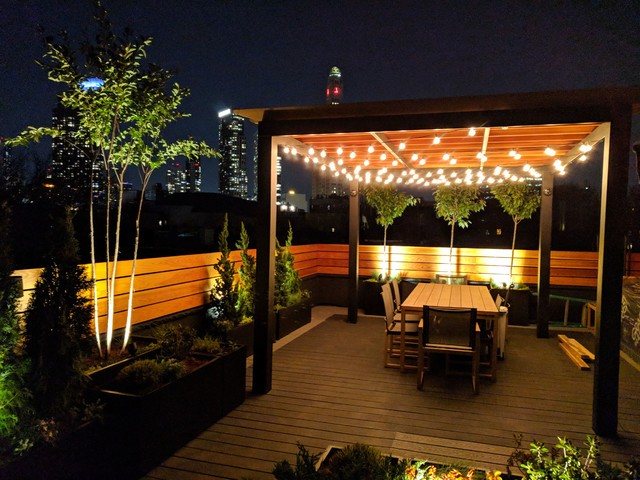The photograph captures a night-time scene on a rooftop deck in a city, illuminated by the soft glow of skyscrapers lighting up the dark sky. The deck, with its wooden panels and rails, features a central gazebo adorned with hanging lights. Underneath the gazebo, a wooden table and chairs suggest an inviting outdoor dining area. Scattered throughout the deck are various plants, including trees, shrubs, and herbs, adding a touch of greenery. Wooden planks and a ladder in the background hint at ongoing construction. The entire area is encircled by a wooden fence, providing a cozy, enclosed atmosphere amidst the urban landscape.